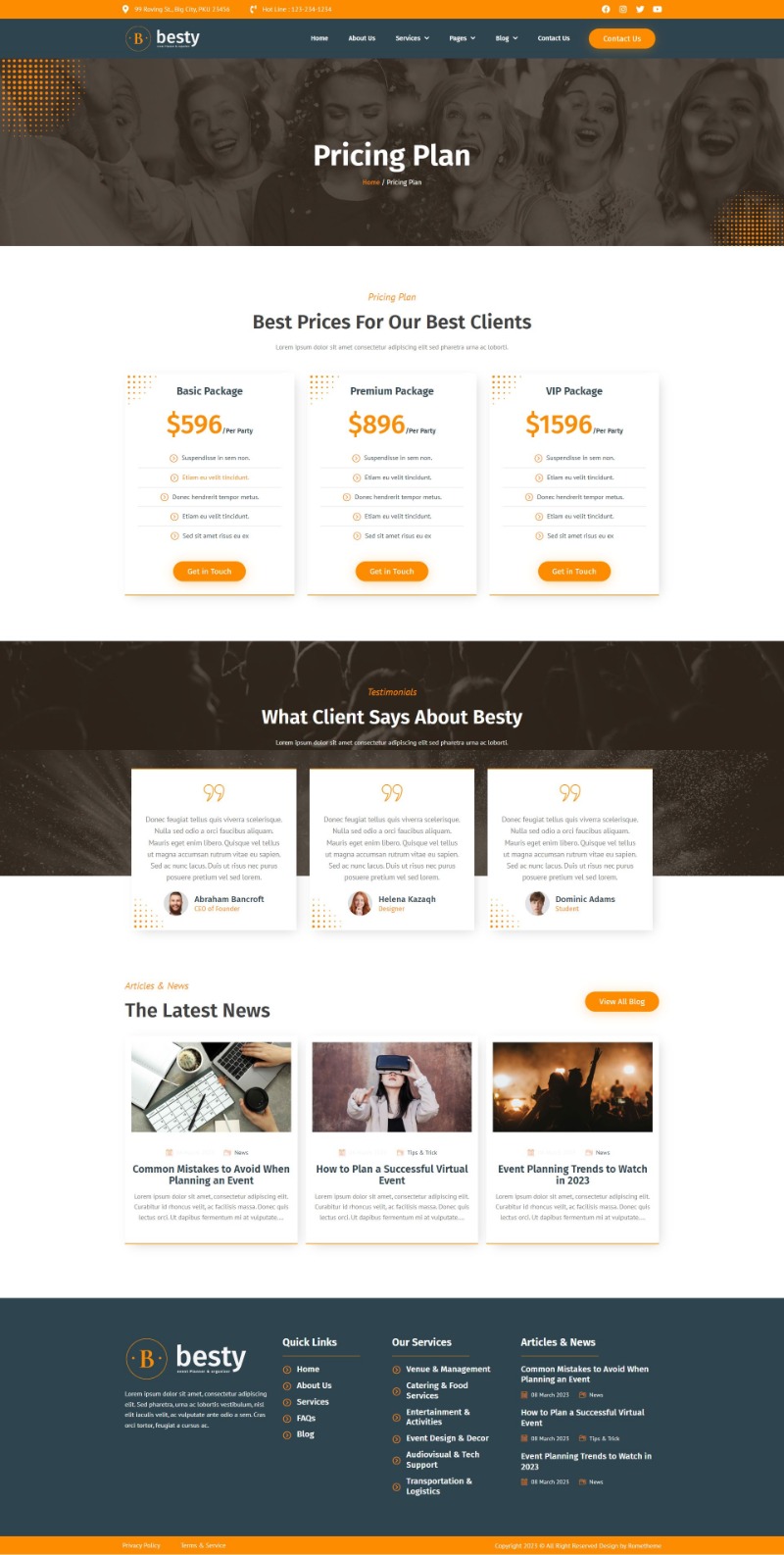The image is a detailed screenshot of a product page from the website of a company named Besty. At the very top of the page, the navigational menu prominently displays the name "Besty". Below that, there is a header with the text "Pricing Plan" written in white against a dark gray background composed of photographs featuring women’s faces. The section beneath the header sports a white background with the tagline "Best prices for our best clients."

Three pricing options are prominently displayed in orange within individual squares, listed from left to right as follows: $596, $896, and $1596. Below this section, a gray banner similar in style to the header graphic appears, featuring the text "What customers say about Besty" in white.

Further down, the page showcases three white squares, which contain client testimonials, although the print is too small to read. Finally, at the bottom of the page, the footer has a grayish-blue background with small, unreadable print, except for the company name "Besty," which stands out in white.